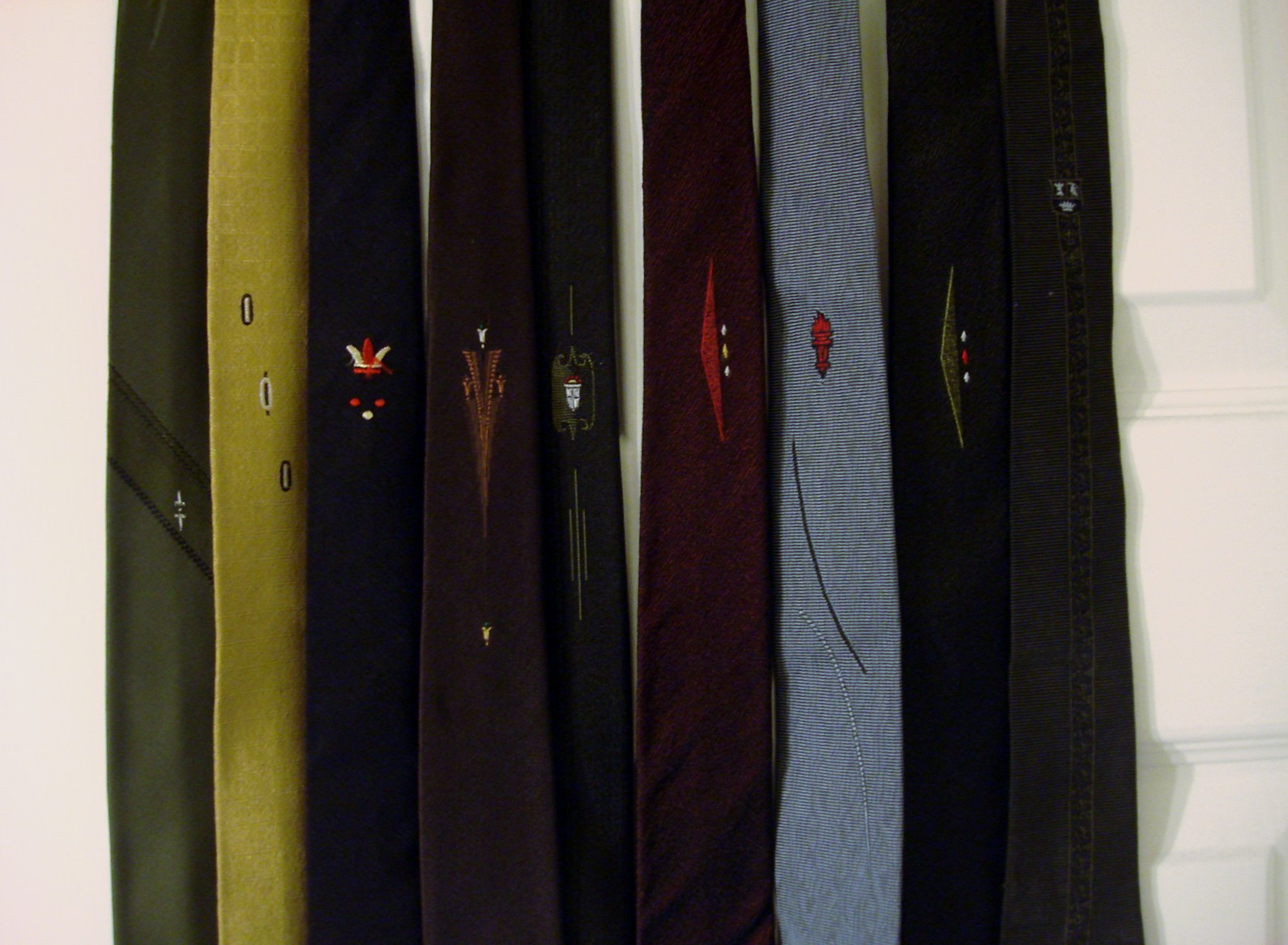The photograph depicts a collection of nine neckties hanging on a hanger with multiple posts, attached to the back of a white, paneled door without a visible door handle. The ties are predominantly dark in color, with individual unique designs and patterns. From left to right, the ties are:

1. Olive green with a small white design featuring two diagonal stripes.
2. Lime green with three small black and white circles.
3. Black featuring a tiny red and white crown-like design.
4. Dark brown with black stripes, adorned with a light brown triangular design in the center.
5. Dark gray displaying a greenish design with a small white and blue crest.
6. Maroon decorated with a red triangle and three white dots.
7. Bluish-white with a prominent red torch design.
8. Black with a small embroidered design consisting of white and red dots.
9. Black with a slightly different shade of black stripe running down the center.

The background consists of a white door, with a section on the right-hand side showing additional lines and rectangular panels, hinting at typical bedroom door features.